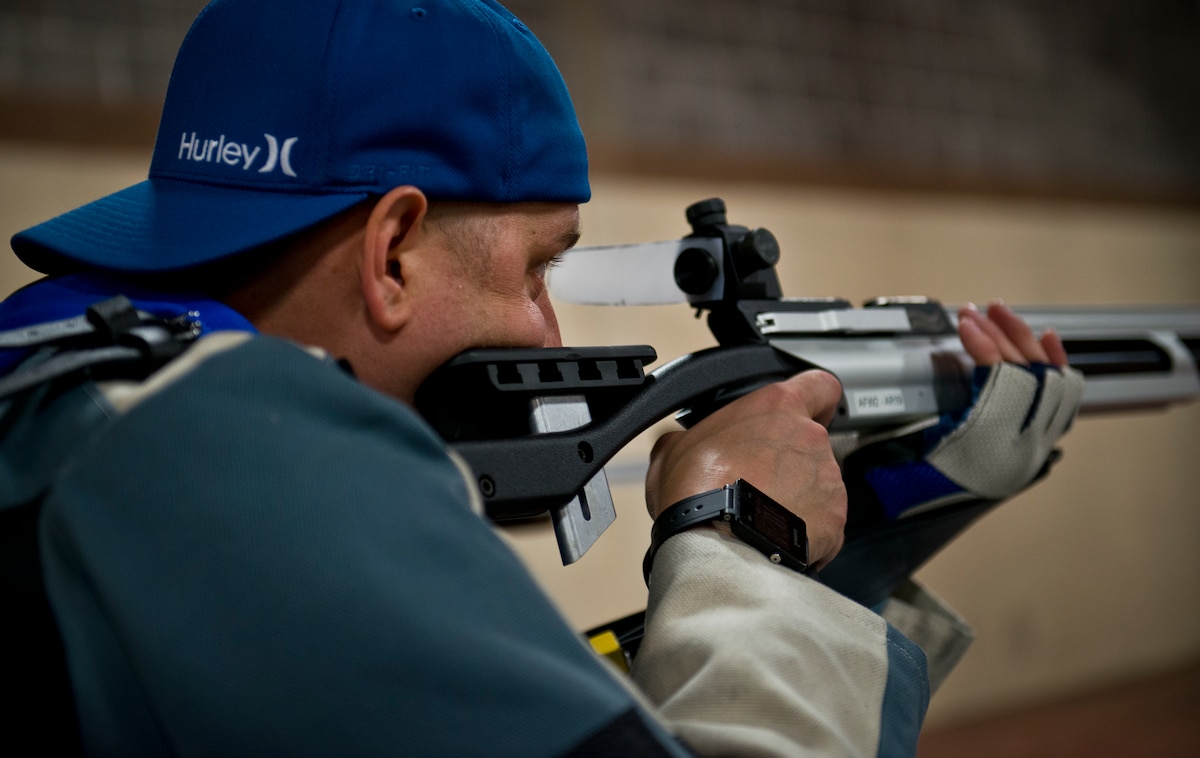A young man is depicted in this detailed photograph, intently shooting a sleek, silver-colored rifle, likely a pellet rifle used in competitive shooting events, such as the Olympics. The rifle is exceptionally detailed, featuring an elaborate black sighting mechanism and an adjustable stock for both cheek rest and length. The barrel is encased in silver shrouds, with brown or black interiors, and additional adjustment mechanisms are visible on the accessories. 

The shooter is dressed in a multi-colored jacket, combining white and dark aqua hues, and wears a blue Hurley cap turned backward. There is an additional blue item partially visible behind his neck. His focused demeanor is emphasized by the precise grip on the rifle, with his trigger finger poised and his other hand stabilizing the front end. A black LCD watch adorns his wrist, further signifying his preparedness. 

The background of the image is blurred, blending beige and hints of gray brick, ensuring that the main focus remains on the marksman and his sophisticated rifle. The overall composition of the photograph, which is longer in width than height, captures a moment of intense concentration and precision in target shooting.